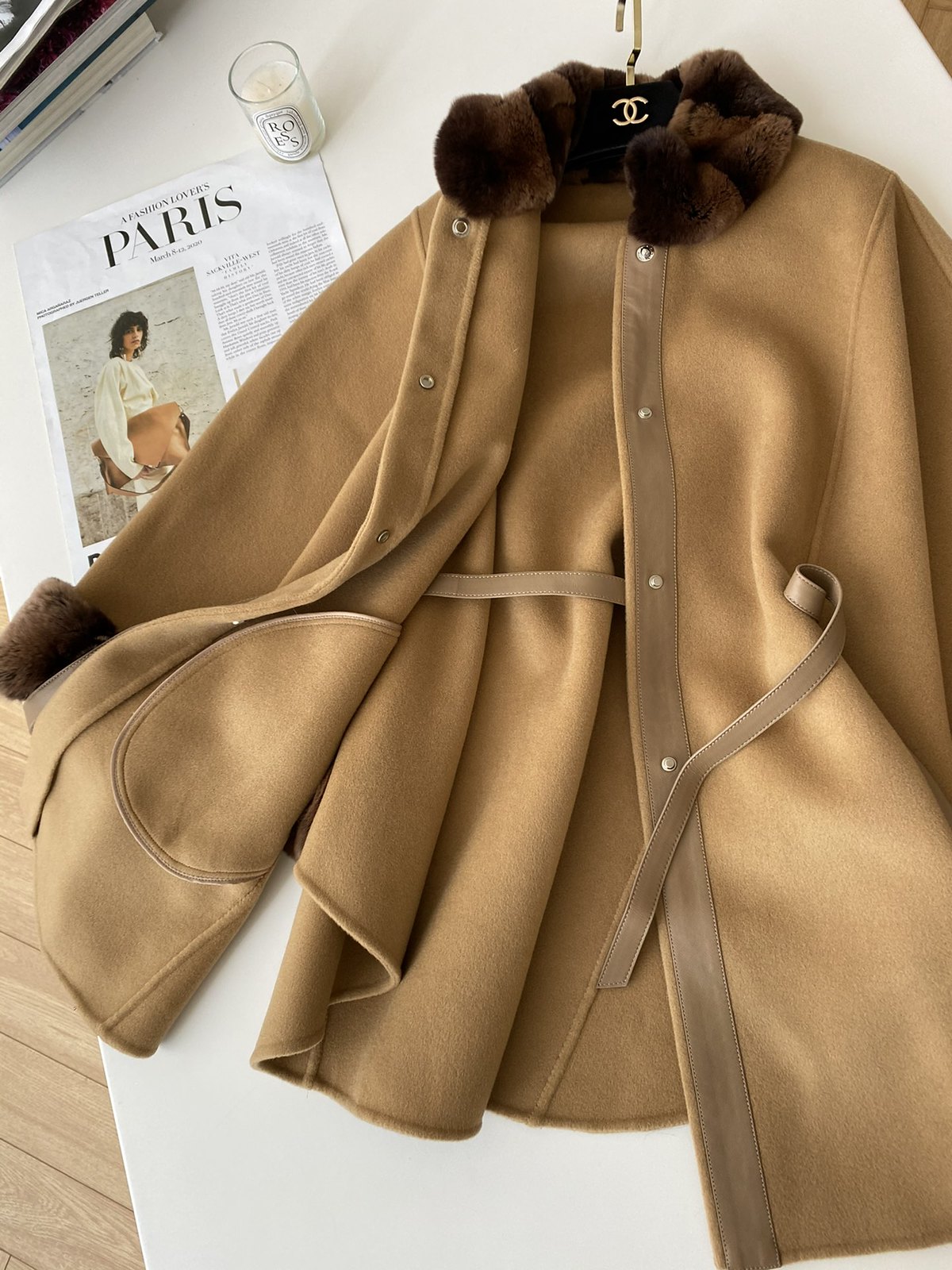This image prominently features a high-end Chanel coat carefully laid upon a white table. The coat, distinguished by its light tan color with darker brown fur accents on the collar and sleeves, exudes luxury and sophistication. It features a golden hanger adorned with the iconic Chanel logo. The coat is designed with a belt that wraps around the waist and several buttons lining the front, adding to its elegant appeal. 

Accompanying the coat on the table is a white candle in a clear glass holder labeled "Roses," adding a touch of subtle ambiance. To the side, there is a magazine or loose-leaf article titled "A Fashion Lover's Paris," featuring an image of a woman, which complements the high-fashion theme. In the background, a few books are neatly stacked, contributing to the photograph's stylish atmosphere and focalizing the luxurious Chanel jacket.